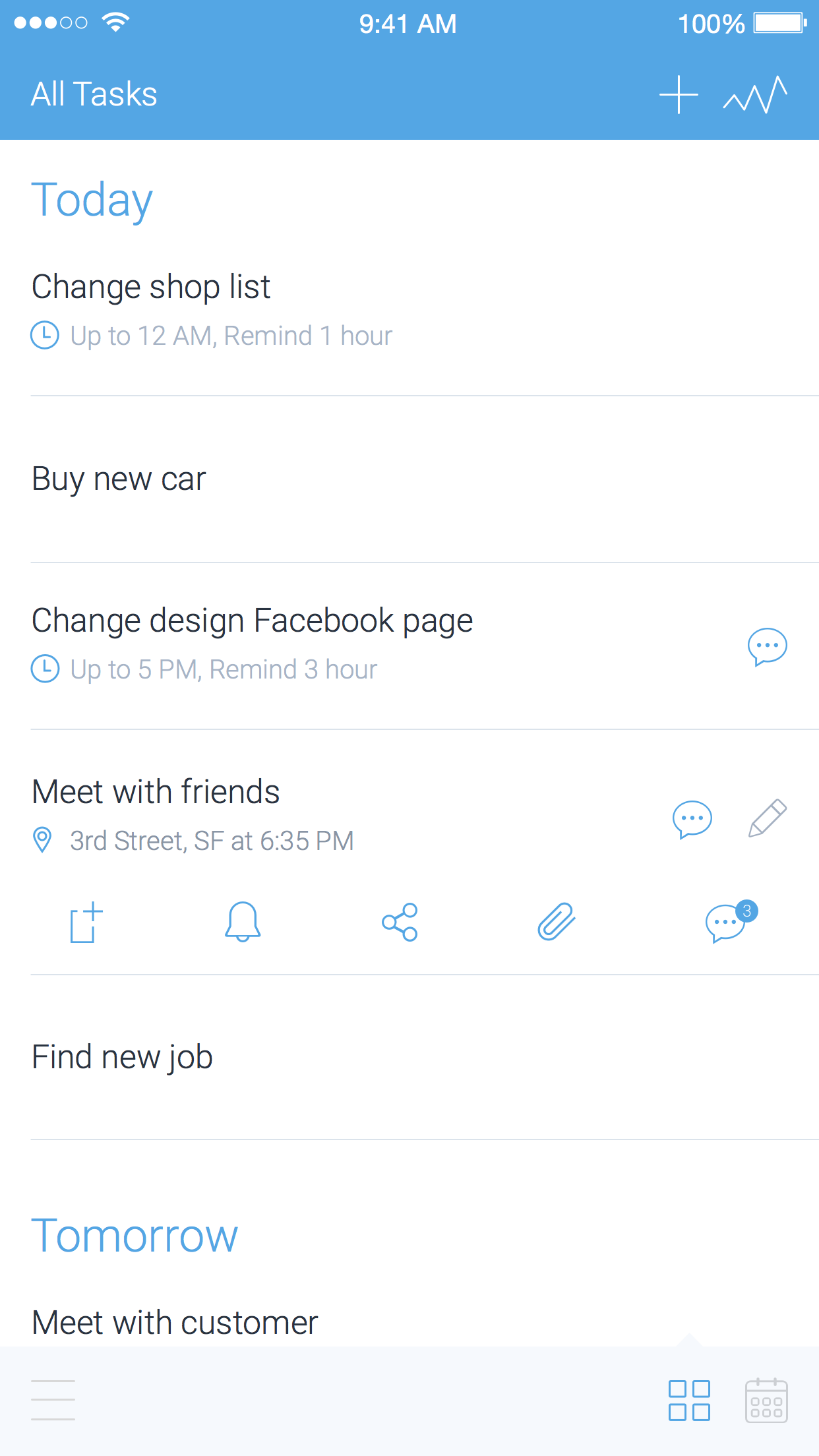The screenshot portrays a meticulously organized to-do list on a smartphone interface, featuring a white background for clear readability.

- **Top Section**:
  - Occupying the top of the screen is a blue triangular rectangle with white text.
  - In the upper left, there are five circles: three are white, and two are blue with white outlines, positioned next to a Wi-Fi signal icon.
  - Below this, bold white text states "All Tasks."

- **Header Info**:
  - **Top Center**: The current time, "9:41 AM," is prominently displayed.
  - **Upper Right Corner**: The battery status reads "100%" with a corresponding battery indicator. Adjacent are two icons: a white "T" and a white graph symbolizing upward progress.

- **Tasks for Today**:
  - In blue text, the word "Today" stands out.
  - Below this, a few tasks are listed with specific details:
    - **Change Shop List**:
      - An analog clock icon indicates a deadline of "Up to 12 AM," with a reminder set for 1 hour prior.
    - **Buy New Car**
    - **Change Design Facebook Page**:
      - Another analog clock shows "Up to 5 PM," with a 3-hour reminder.
    - **Meet with Friends**:
      - Location specified as "3rd Street SF at 6:35 PM."
    - **Find New Job**

- **Tasks for Tomorrow**:
  - In blue text: "Tomorrow."
  - One listed task:
    - **Meet with Customer**

The format and color coding enhance the functionality and intuitiveness of the to-do list, ensuring that the user can easily manage and prioritize their daily and upcoming tasks.